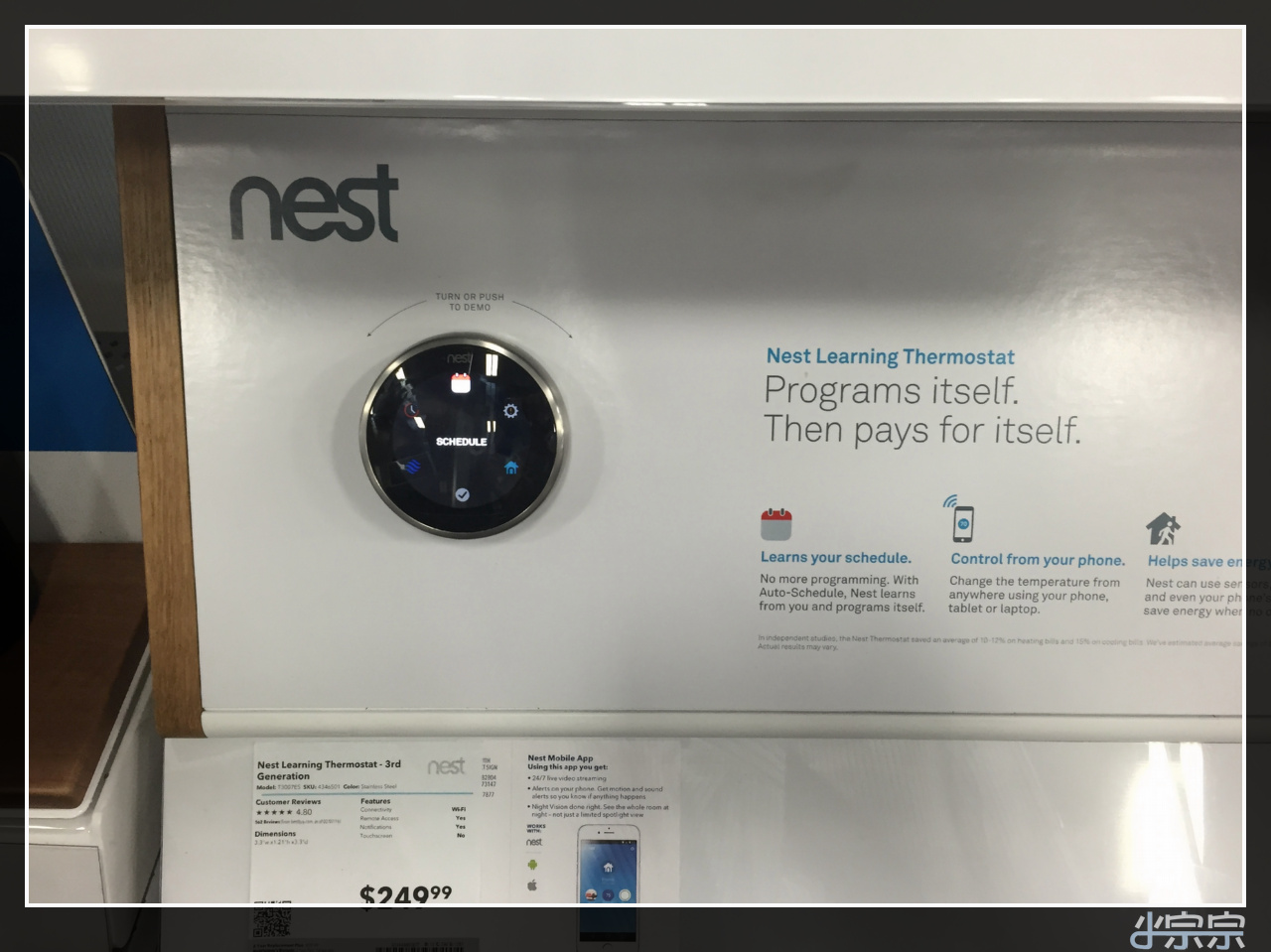This photograph captures a sleek, modern Nest Learning Thermostat prominently displayed in a retail store. The thermostat, a round device with an LED digital readout, is showcased on a display board to the right. The digital screen on the thermostat showcases its innovative features. Positioned below the display board, the partially visible product tag reveals the price, listed at $249.99. The display board highlights key selling points, stating, "Nest Learning Thermostat: Programs itself, then pays for itself." Although additional information is present below this statement, it is rendered illegible due to its small size in the photograph.